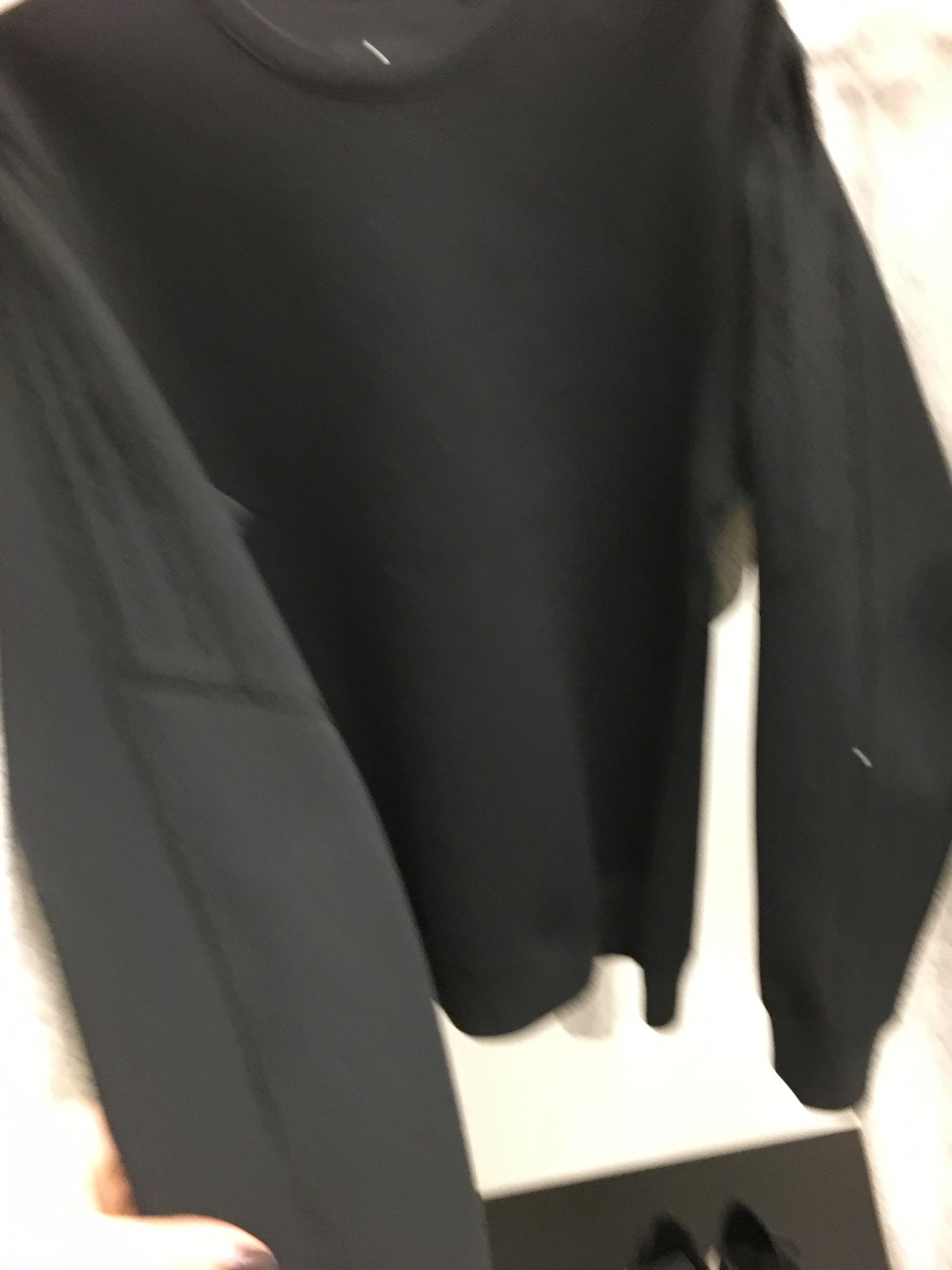The image depicts a close-up of a loose, black sweatshirt with long sleeves that feature distinctive embroidered lines; one line runs vertically down the sleeve while another runs perpendicularly. The sweatshirt seems to have a circular collar and a small white label around it. In the lower left-hand corner of the photograph, a person's thumb with brown nail polish peeks in, suggesting they are holding the sleeve of the sweatshirt to examine it. A part of the white wall occupies the background, while the bottom of the image shows what appears to be a partially visible black square with elements that may be footwear, though they are cut off and indistinguishable. Despite the image’s blurriness, details like the white dot on the sleeve and another near the top of the shirt are noticeable. Additionally, a gray sleeve with darker indents, likely from another garment, is faintly visible to the left, reinforcing the impression that the scene might be inside a shop where multiple clothes are being browsed.